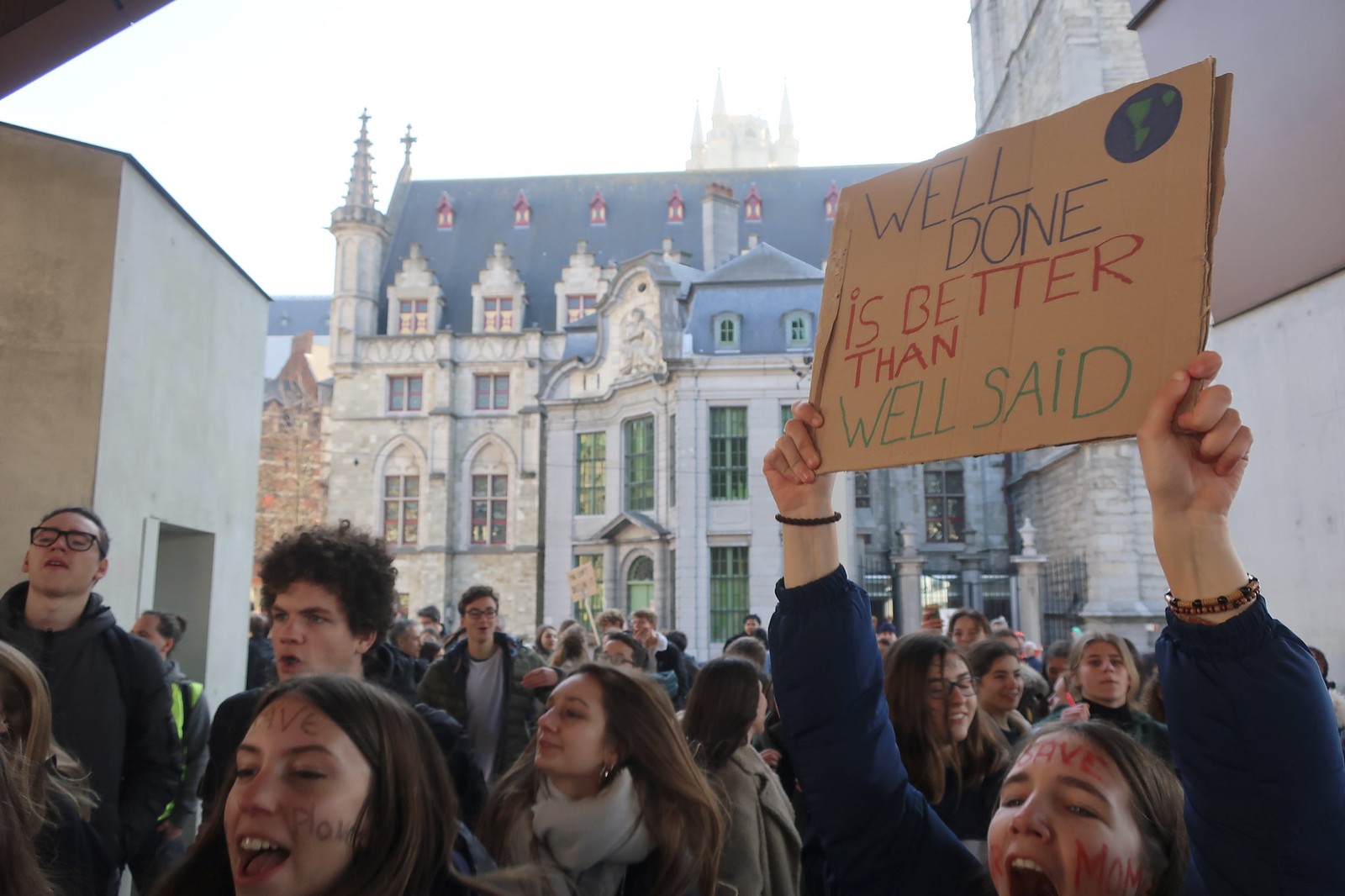In a bustling European city, a vibrant protest unfolds against the backdrop of a majestic 16th or 17th-century building adorned with spires, turrets, and a steep roof, reminiscent of a medieval castle or cathedral. The absence of cars on the cobblestone street underscores the historical ambiance of the scene. At the forefront stand two young women with dark brown hair, both fervently engaged in the protest, having painted words on their faces. The woman on the left has "SAVE" on her forehead and "LOVE" on her cheek, while the woman on the right, possibly shouting a chant, has "SAVE" on her forehead and additional, unidentifiable lettering on her cheeks.

The woman on the right prominently holds a homemade sign, intricately designed with multi-colored uppercase letters proclaiming, "WELL DONE IS BETTER THAN WELL SAID." The phrase "WELL DONE" is in blue, "IS BETTER THAN" in red, and "WELL SAID" in green, accompanied by an image of the globe on the top right corner. This young, diverse crowd, numbering around fifty, consisting of an equal mix of males and females, many donning winter coats and scarves, channels their collective energy into the cause they champion, standing united in front of this storied and symbolic architecture.